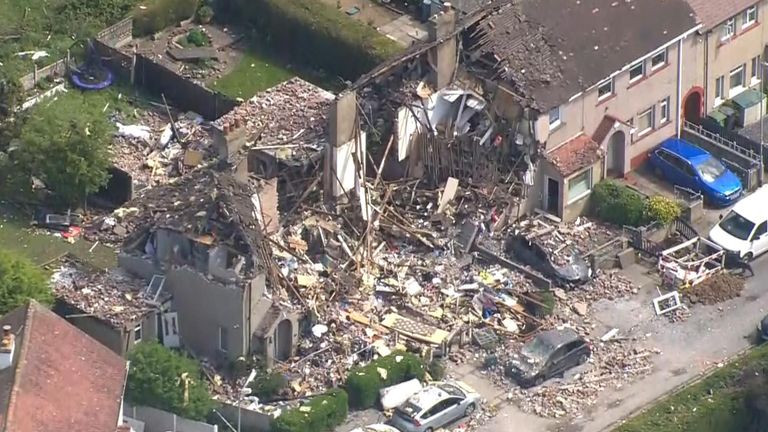This aerial photo depicts the aftermath of a catastrophic event that has left a house almost entirely demolished. The building is reduced to rubble, with debris strewn across the ground, covering three nearby cars. Another residence adjacent to the destroyed house has minor roof damage but remains largely intact. This intact neighboring house, a beige apartment, has visible windows and a red archway. To its side, there is a driveway with a blue van parked, while a white van is parked in another driveway nearby. Between these homes, a black fence and several dumpsters can be seen. In the backyard of the demolished house, green grass, hedges, trees, and a trampoline are visible, indicating it's daytime due to the bright conditions. The overall scene suggests a severe, unplanned incident—potentially a bombing or natural disaster. The architectural style hints that this could be in Europe, with the cars appearing modern, indicating the photo was taken within the last 10 to 20 years.